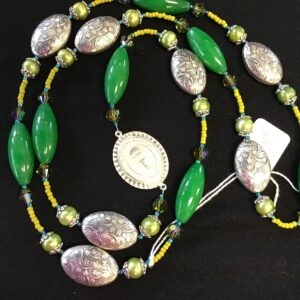The image displays a meticulously crafted beaded necklace set against a pure black background. Central to the design is a metallic, coin-shaped medallion with ribbed edges, exuding a bright, silver-like sheen. The necklace features a harmonious arrangement of various beads: large, elongated green beads reminiscent of pebbles; small, vibrant yellow beads; round golden beads; and further intricate beads with hues of off-white and pink, some engraved with delicate flower designs. The pattern of these beads alternates and spirals outward, creating a mesmerizing visual rhythm. Additionally, a delicate white string is tied to one end of the necklace, affixed with a small white tag that potentially carries information about the piece. The necklace itself appears to be gently coiled atop the black surface, enhancing its intricate details and craftsmanship.